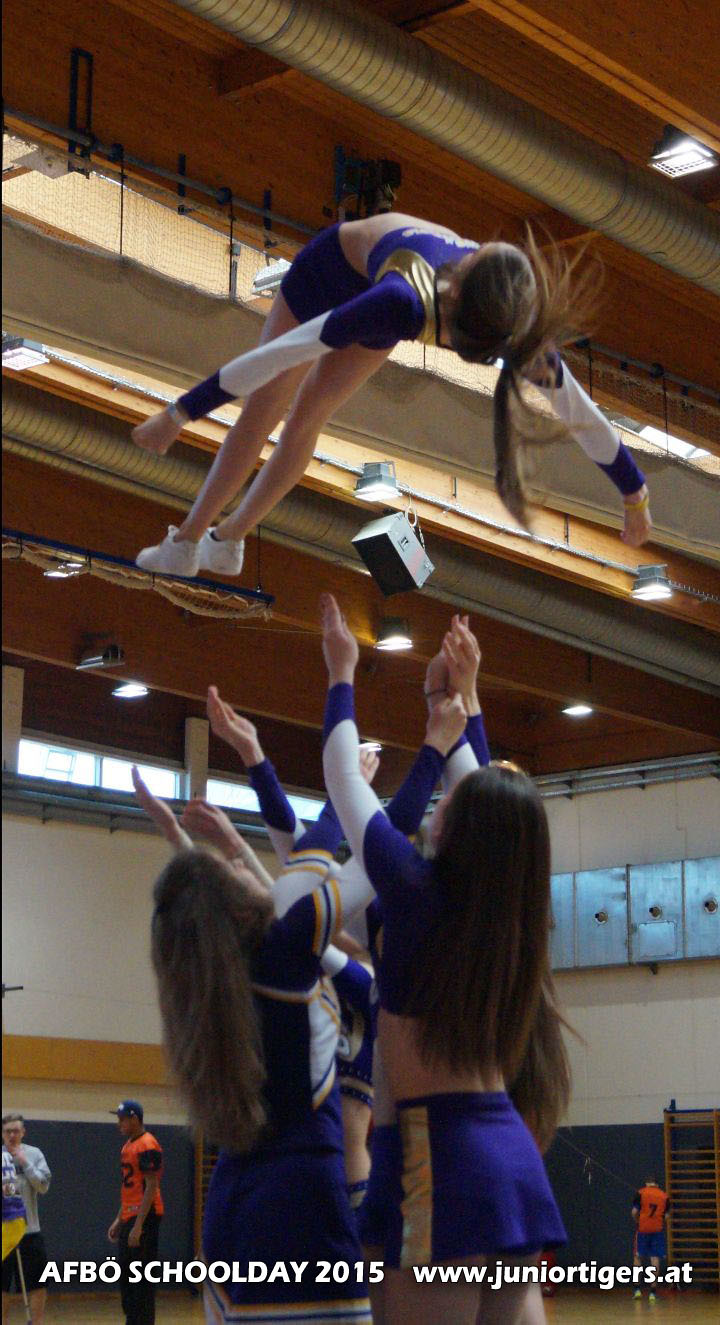This photograph, taken inside a gymnasium with high ceilings and visible stands, captures an exhilarating moment during a cheerleading performance. At the center, four cheerleaders in purple and gold skirts and tops stand chest to chest in a circle with their arms stretched upwards. They are in the process of catching a fifth cheerleader who has been tossed into the air. This cheerleader is about four to five feet above them, with her back arched, facing upward, her legs stretched out together, and her arms out to the sides in a capital T position. Her hair is flying around as she descends towards her teammates. In the background, two sports team members in identical orange jerseys, one numbered seven, and a few other individuals, including a coach or an adult, can be seen. The image is captioned at the bottom with the text "Off Bow School Day 2015 www.juniortigers.at."